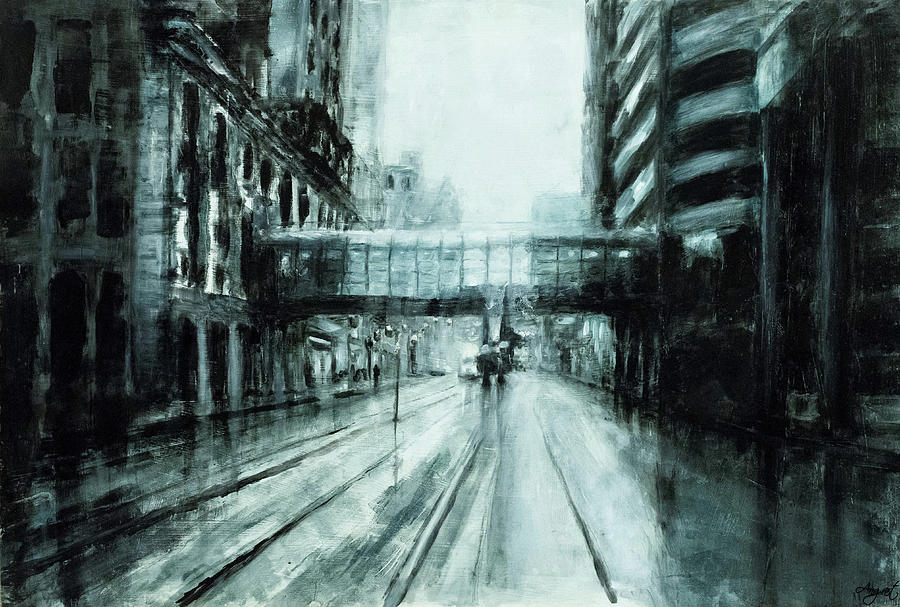This detailed pencil drawing depicts a city street scene with a slight off-center perspective, focused on the inside left lane of a four-lane road. Approximately half a block ahead, a covered, see-through plexiglass or glass catwalk spans across the street, connecting buildings on either side. The buildings beyond the catwalk lack intricate detail, adding to the drawing's overall grayish tint. Underneath the catwalk, where it is supported by a beam on the street, stand two or three indistinct figures. Despite the lack of color, the drawing suggests a daytime setting through the presence of light rendered above the scene.